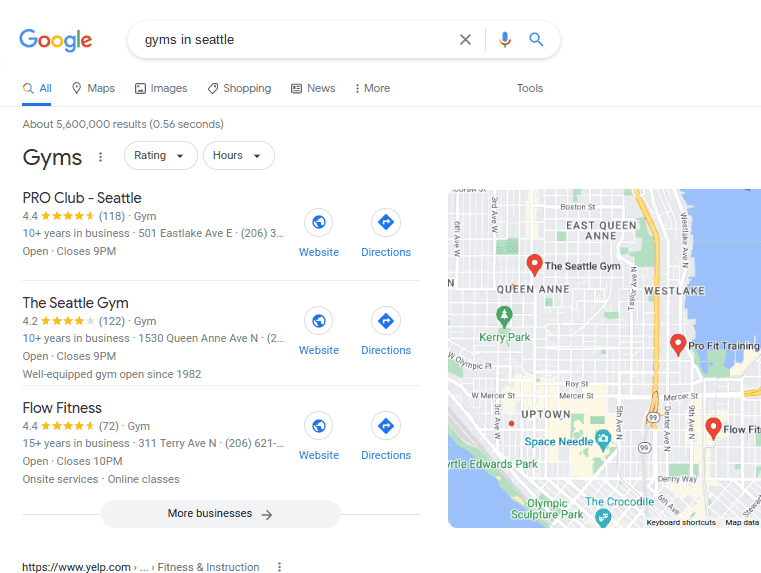This image appears to be a screenshot of a computer displaying a Google search results page. The background is white with the Google logo prominently displayed in blue, red, yellow, and green colors in the upper left corner. To the right of the logo is a search bar with the query "gyms in Seattle" typed in. Below the search bar are filter options including "All," "Maps," "Images," "Shopping," "News," and "More," with a blue underline highlighting "All."

The search results indicate approximately 5,600,000 results. Displayed prominently underneath are three gym options, along with a map to the right that shows drop pins for their locations. The first gym listed is "Pro Club in Seattle," boasting a 4.4-star rating with the stars colored yellow. Information for the gym includes links to its website and directions. The second listing is "Seattle Gym," with a 4.2-star rating, also providing links to the website and directions. The third gym, "Flow Fitness," has a 4.4-star rating and similarly includes website and directions links.